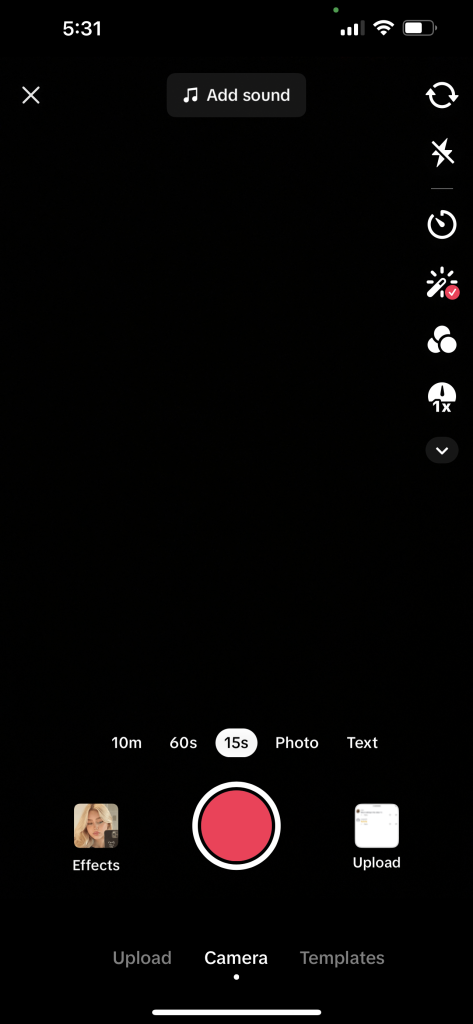This is an intricately detailed screenshot of a mobile device in its camera app interface. In the top left corner, the time is displayed as 5:31. Moving to the top right, the screen shows icons for cell signal, Wi-Fi, and battery status.

Below the time, a white 'X' icon allows the user to exit the screen. Next to the 'X', centered at the top, there is an option to "Add Sound". On the right side of the display, the screen features a refresh or rotate symbol followed by icons for flash and four more settings icons that allow adjustments and effects to be applied to photos or videos.

Below these icons, a timer is available with options for 10 minutes, 60 seconds, and 15 seconds. Further down, there are text options labeled "Photo", and an "Effects" button in the bottom left.

Located centrally at the bottom is a prominent red button used for recording or taking a photo. The bottom right corner has an "Upload" button, and below the red button, options for "Upload", "Camera", and "Templates" are displayed.